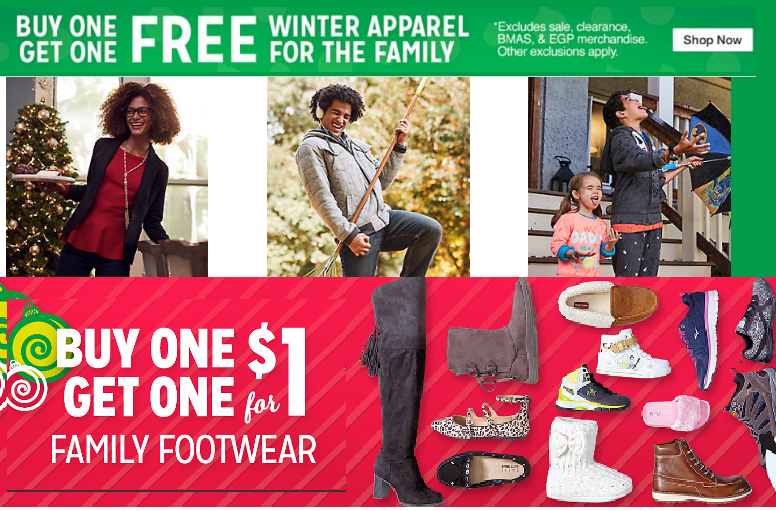The advertisement features a green header with a prominent message in white capital letters that reads, "BUY ONE GET ONE FREE WINTER APPAREL FOR THE FAMILY." Beneath that, in smaller text, the message clarifies that exclusions apply, mentioning, "Excludes sales clearance, B.M.A.S. and E.G.P. merchandise. Other exclusions apply." A white rectangular button below this text says, "Shop Now."

On the left side of the ad, there's an image of a woman dressed in a red shirt and a black suit jacket, standing next to a Christmas tree adorned with gold ornaments. To her right, a man wearing headphones and a gray jacket holds a rake posed like a guitar, adding a whimsical touch to the scene. Below these figures, two kids are seen standing on steps, adding a familial and festive feel to the advertisement.

Towards the bottom of the ad, a pink box with text states, "BUY ONE GET ONE FOR ONE DOLLAR FAMILY FOOTWEAR." Beside this box, there is an illustration of Christmas ornaments on the left and a display of various footwear, including shoes, boots, flip-flops, and casual sneakers, on the right. This detailed depiction creates a vivid and festive promotional image for winter apparel and footwear.